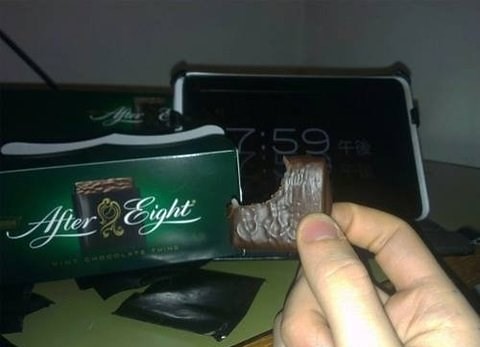The image is a color photo captured in landscape orientation, showcasing a hand with slender fingers holding a partially eaten square of After Eight chocolate mint. The setting appears dark, with the flash from the camera providing illumination. In the background, slightly out of focus, is a green box that resembles a tea bag package, detailed with elegant white script spelling "After Eight." The box also features an image of the individually wrapped chocolates in dark brown sleeves, some of which are scattered empty on the desktop. A digital clock displaying "7:59 PM" adds a humorous touch, as it is not yet after eight o'clock. The scene includes a dark gray wall, enhancing the sophisticated feel of this snapshot of gourmet candy.